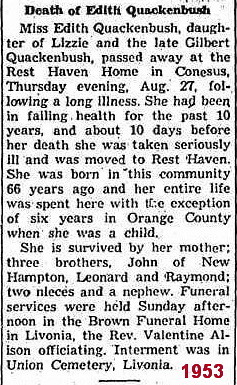The image shows an excerpt from a newspaper article, set against a white background with black text, detailing the death of Edith Quackenbush. The headline, in bold serif font, reads "Death of Edith Quackenbush." Directly beneath, in the same font size but not bolded, it states, "Miss Edith Quackenbush, daughter of Lizzie and the late Gilbert Quackenbush, passed away at the Rest Haven home in Canisius Thursday evening, August 27, following a long illness." The article continues to elaborate that Edith had been in failing health for the past 10 years and became seriously ill 10 days before her death, prompting her move to Rest Haven. She was born in this community 66 years ago and spent her entire life here, except for six years in Orange County during her childhood. Edith is survived by her mother, three brothers (John of New Hampton, Leonard, and Raymond), two nieces, and a nephew. Funeral services were held Sunday afternoon at the Brown Funeral Home in Livonia, with Reverend Valentine Allison officiating. Interment was in Union Cemetery, Livonia. A distinct feature of the image is the year "1953" in red sans-serif font at the bottom right corner, contrasting the rest of the serif font text. The article is framed by vertical lines on both the left and right sides running the full length of the text.